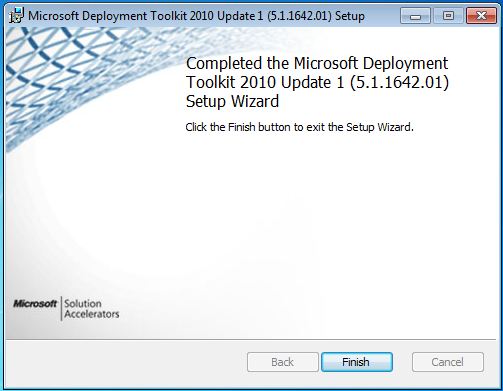The image captures the final screen of the Microsoft Deployment Toolkit 2010 Update 1 Setup Wizard, specifically version 5.1.1642.01, as seen on a Windows operating system, likely Windows Vista or Windows 7. The window prominently displays confirmation text stating that the setup wizard has been completed, with instructions to click the Finish button to exit. The setup window features familiar Windows UI elements, including the Minimize, Maximize, and Close (red X) buttons at the top right corner. The window title bar is in blue, highlighting the application name. At the bottom left of the window, the text "Microsoft Solution Accelerators" is visible, alongside interactive buttons labeled Back, Finish, and Cancel, providing navigation options for the user.